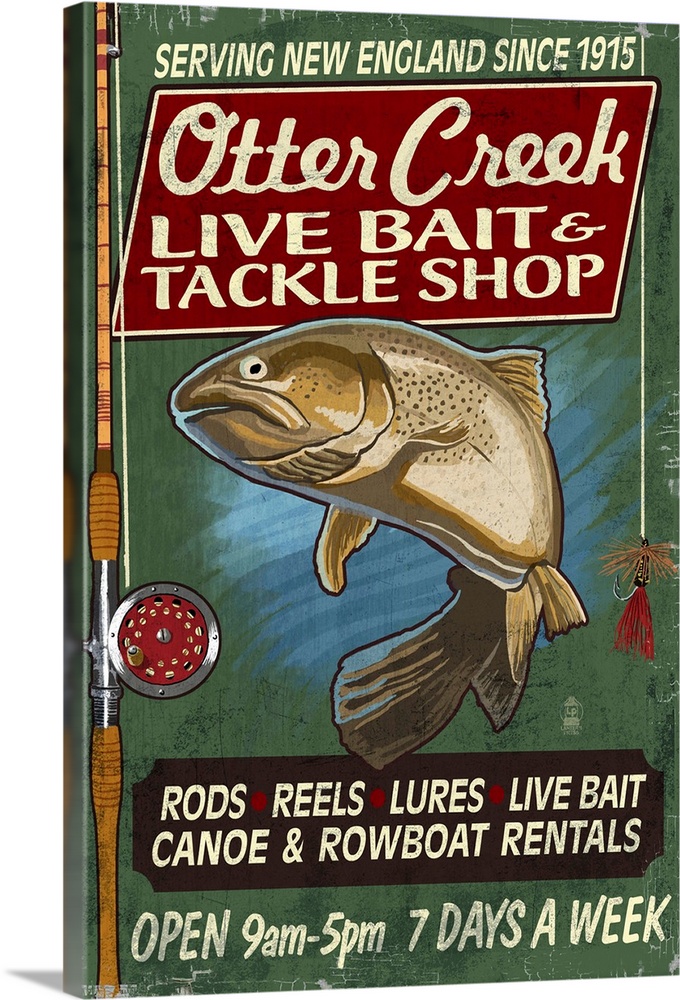The image features a vintage-style painted sign with an ornate and colorful design. At the top, white text on a green background reads, "Serving New England since 1915." Below this, a red parallelogram with a white outline contains the text "Otter Creek Live Bait and Tackle Shop" in a mix of cursive and regular fonts. Dominating the center of the image is a large, brownish-white fish against the green background. To the left, a fishing rod with a yellow-gold tint and a red and silver reel extends upward, with the line arcing down towards a lure and hook featuring red and yellow elements. Beneath the fish, a black banner with white text and red circles spells out: "Rods, Reels, Lures, Live Bait," and "Canoe and Rowboat Rentals." At the very bottom, additional text on the green background states, "Open 9 a.m. to 5 p.m. seven days a week." The sign, which resembles a cartoon or wooden painting, stands against a plain white backdrop, emphasizing its detailed, vibrant design.